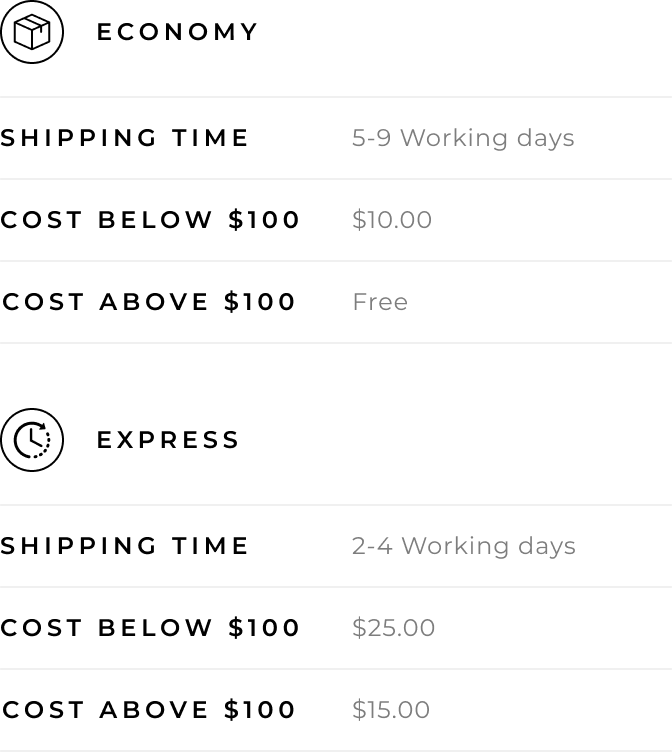This image is a screenshot of a website, set against a white background. In the upper left corner, there is a black circle containing an icon of a package. To the right of this icon, the word "Economy" is written in black font. Below it, a black horizontal line separates the sections.

The next section details shipping options. It starts with the text "Shipping Time" in black font, followed by "5 to 9 working days" in gray font. Below this, it states "Cost below $100" in black font with the amount "$10" in gray font, and then "Cost above $100" in black font with "Free" in gray font beneath it.

The second section is identified by the word "Express" in black font, accompanied by a circle icon featuring a clock, positioned to the left. Directly below this icon, "Shipping Time" is again written in black font, followed by "2-4 working days" in gray font. The cost details are outlined next: "Cost below $100" in black font with "$25" in gray font, and "Cost above $100" in black font accompanied by "$15" in gray font. Below this section is a faint black line. 

The layout is clean, with clearly differentiated sections and fonts, effectively presenting the shipping options and associated costs for economic and express delivery services.